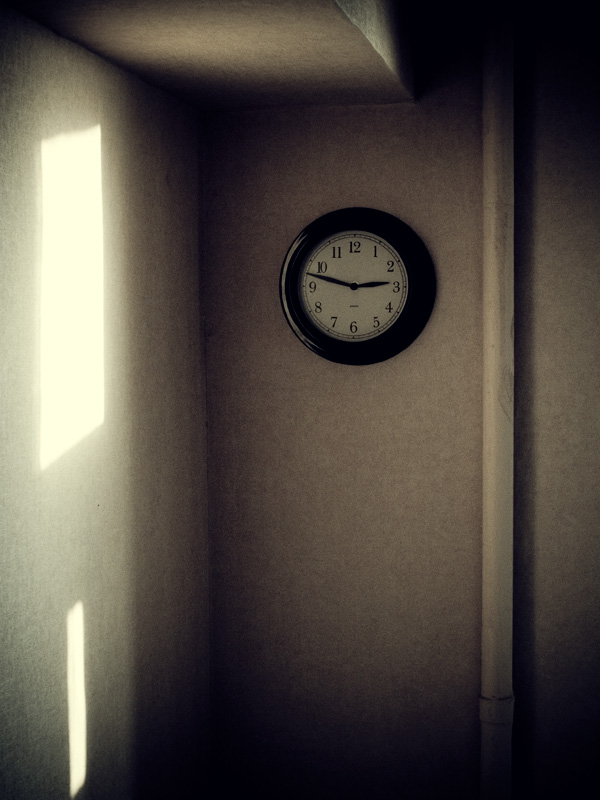This is a detailed photograph of a wall-mounted analog clock positioned near the corner of a room. The clock has a thick black casing surrounding a white face with black Arabic numerals from 1 to 12. The time displayed is approximately 2:47, with the hour hand near 3 and the minute hand between 9 and 10. To the right of the clock, a white downpipe runs vertically along the wall. Above the clock is a white bulkhead. The corner of the room appears to the left of the clock, where light from an unseen window casts a bright rectangular pattern on the adjacent wall, contributing to the black-and-white feel of the image, likely due to a filter. Shadows from the window without shades are visible, enhancing the overall contrast.